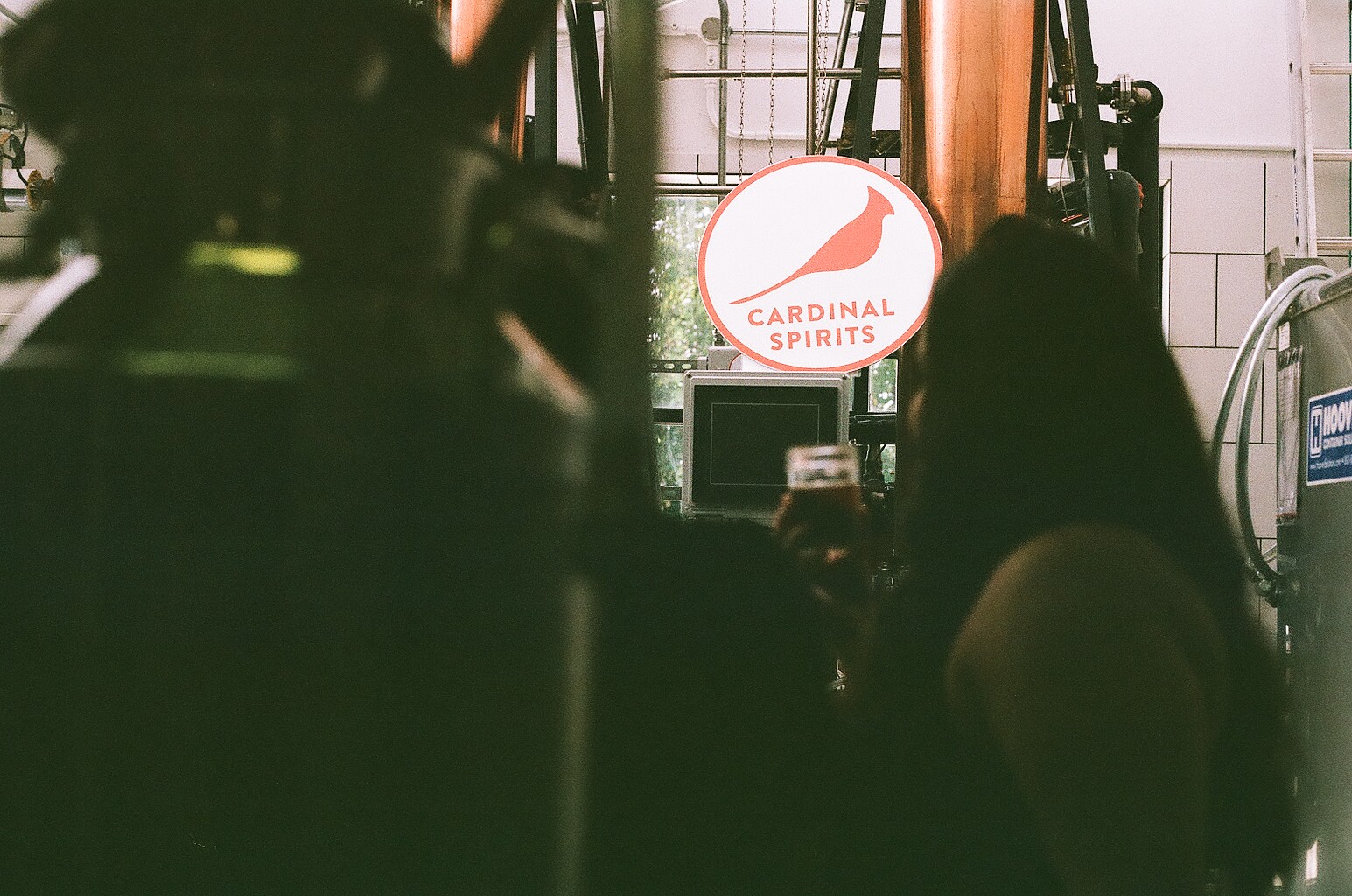In this image tinted with a greenish hue, a woman is prominently positioned in the lower right corner, within what seems to be a factory or distillery setting. The woman, who is wearing a tank top, faces left, displaying her thick arm while her thick, dark hair partially obscures her face, revealing only her cheek and forehead. She holds a small glass filled with a brown liquid in her extended hand. The background features a white tile wall with a white ladder in the upper right corner, and a prominent metallic machine is seen beside her, partially covered by a blue sign that reads "HOOV." To the left, an orange pole stands next to a circular white sign adorned with a red illustration of a cardinal and the red-lettered text "Cardinal Spirits." The industrial ambiance combined with detailed elements suggests the woman might be sampling a drink produced at the facility, possibly a distillery or brewery.